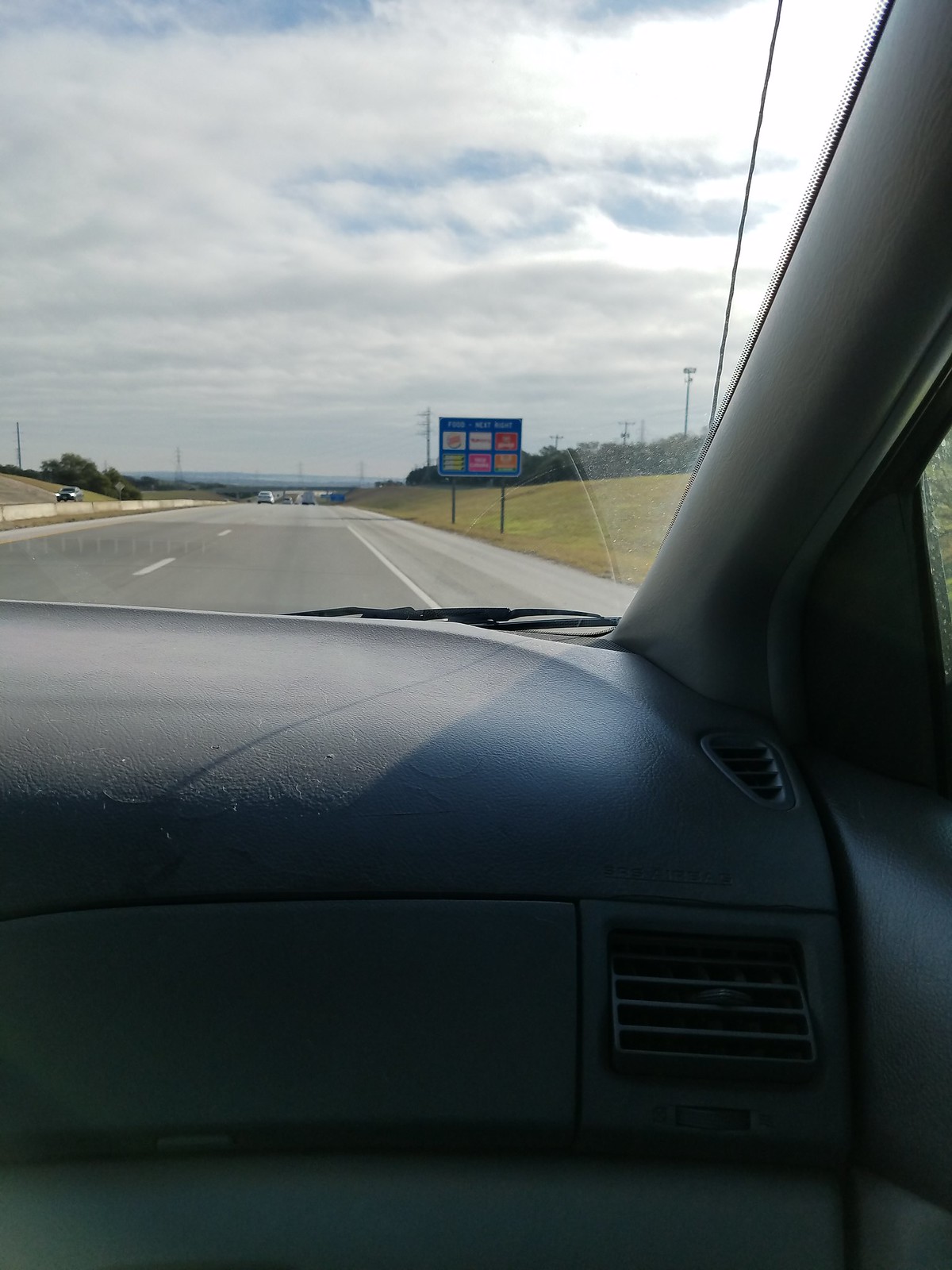A detailed photograph captured from the interior of a car, through the windshield, showcases a dusty gray dashboard at the bottom edge of the image. The windshield itself is partially obscured by a black wiper blade, which has cleared an arched path through an otherwise dusty and frosted surface, leaving a stark contrast between the clean and uncleaned areas. Beyond the windshield, a blacktop highway with white divider lines stretches ahead, bordered by patches of greenish-brown grass on either side. A cement median separates the lanes of oncoming traffic. Off to the right, a blue highway sign indicates a rest stop featuring Burger King, Subway, and other restaurants. Above the scene, power lines span across the freeway and run parallel to it, beneath a mostly cloudy sky with occasional glimpses of blue.